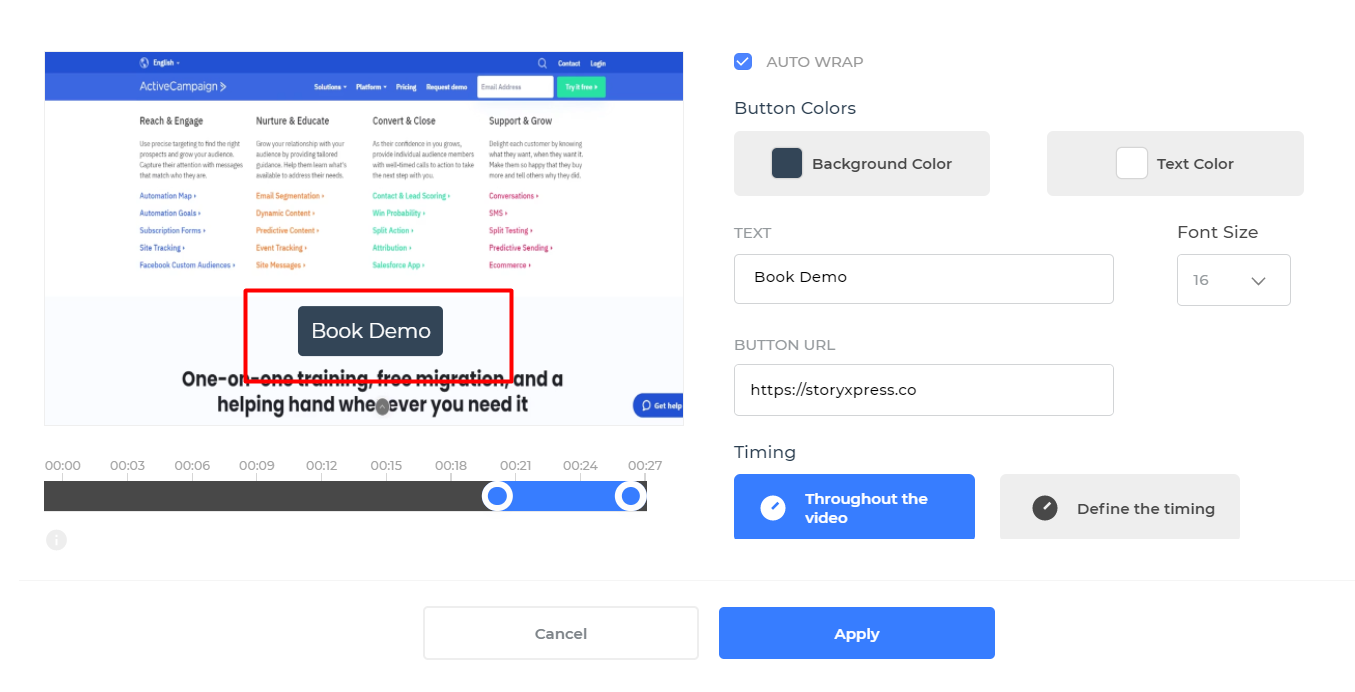The image features a screenshot of a website, likely part of a presentation showcasing a book demo section. 

At the top of the webpage, a blue navigation bar is visible, with options for changing the language (defaulting to English) represented by a globe icon. Following this, there are links for Search, Contact, and Login. Below these are further navigation options including ActiveCampaign, Solutions, Platform, Pricing, and Request Demo. Additionally, there is a field for entering an email address and a prominent green "Try It Free" button.

The webpage structure is divided into several sections with distinct colors and headings. The first section, titled "Reach and Engage," includes dropdown menus, all text appearing in blue. The next section, "Nurture and Educate," features text in orange. Following this is the "Convert and Close" section, with text in green. Lastly, the "Support and Grow" section has text in pink.

Towards the bottom of the image, there is a highlighted "Book Demo" area, which promises one-on-one training, free migration, and ongoing support. The "Book Demo" text is emphasized by a red rectangle, drawing attention to this critical call-to-action. Additionally, the right side of the image appears zoomed in, likely for easier viewing during a presentation, focusing on this crucial section.